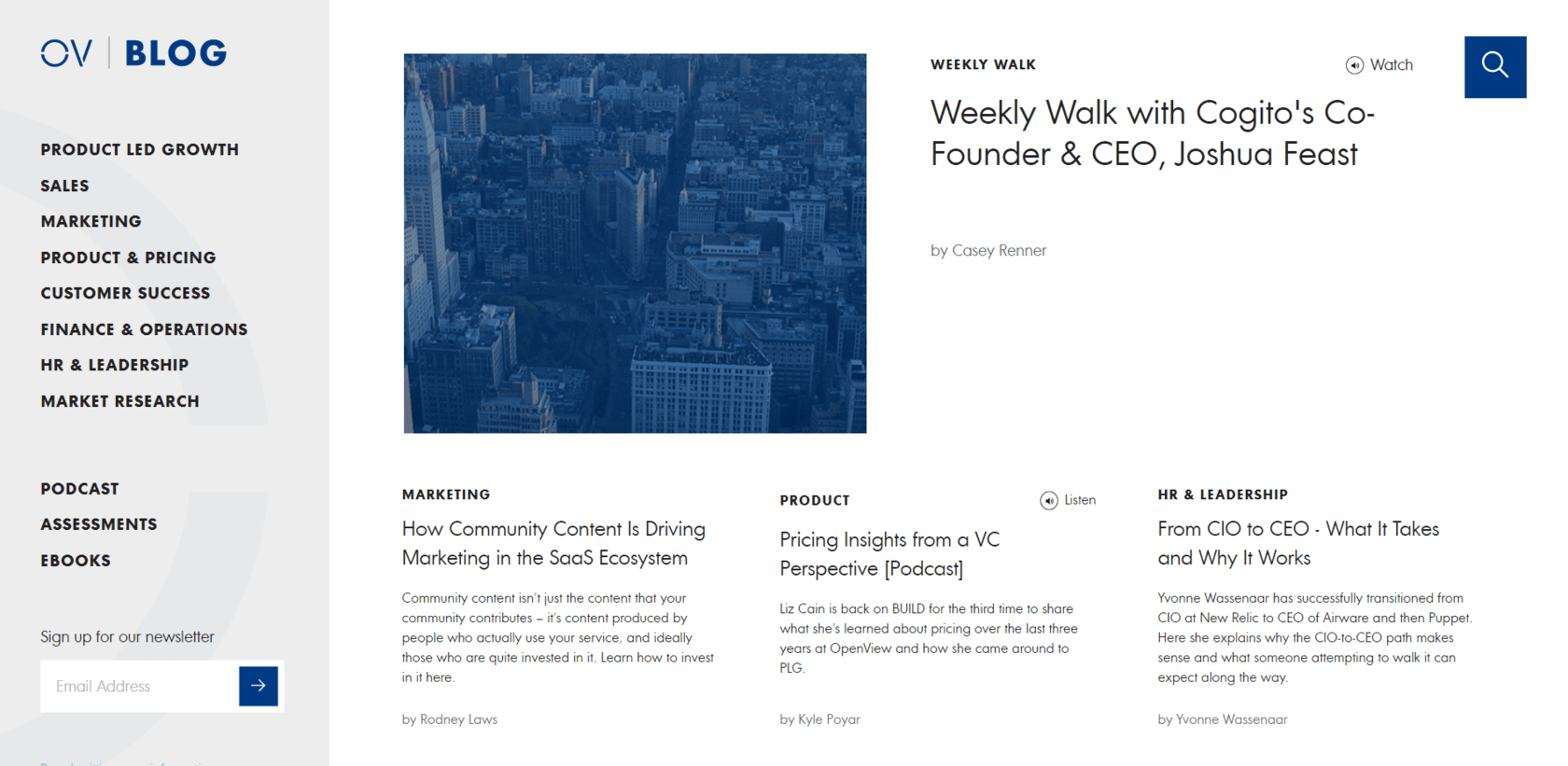**Left Hand Side:**

A vertical blueish-gray rectangle aligns with the left edge of the image, containing various categories and options in blue and black text. The categories are as follows:
- Blue text: "OV-Blog"
- Black text:
  - "Product LED Growth"
  - "Sales, Marketing, Product and Pricing"
  - "Customer Success"
  - "Finance and Operations"
  - "HR and Leadership"
  - "Marketing Research"
- Additional resources in black text:
  - "Podcasts"
  - "Assessments"
  - "E-Books"

At the bottom, there's a gray "Sign up for a newsletter" section with a white input field for entering an email address.

**Right Hand Side:**

A white background features a slightly blurred image of a city skyline at the top. Next to the skyline image, in black text:
- "Weekly Walk" 
- "Watch" with a blue square containing a white magnifying glass icon next to it

Below this section, the text reads:
- "Weekly Walk with Cord George, Co-Founder and CEO Joshua Feist," in black, followed by smaller gray text: "By Casey Rayner"

Underneath this section, a series of articles are listed:

1. **Marketing**
   - **Title:** "How Community Content is Driving Marketing in the SOS Ecosystem"
   - **Description:** (Gray text)

2. **Product**
   - **Title:** "Pricing Insights from a VC Perspective Podcast"
   - **Description:** (Gray text)

3. **HR Leadership**
   - **Title:** "From CIO to CEO: What It Takes and Why It Works"
   - **Description:** (Gray text)